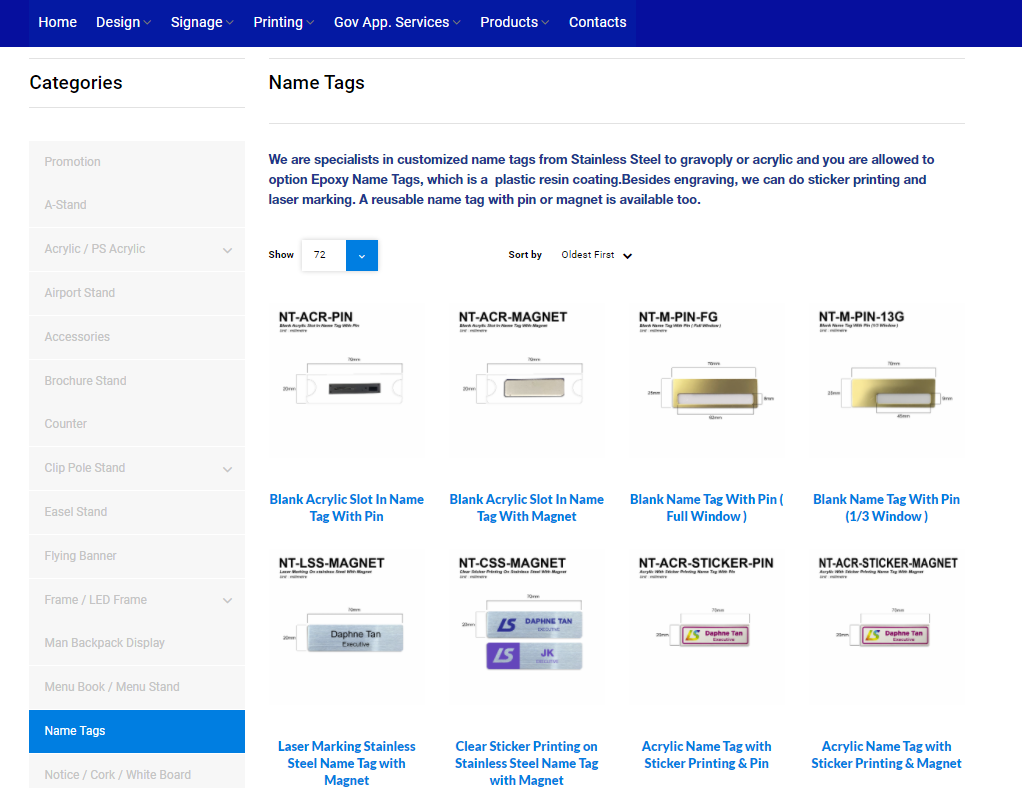The image is a screenshot of a website with a predominantly blue header. The website features a navigational bar with white text, listing tabs such as Home, Design, Signage, Printing, GovApp.Services, Projects, and Contacts. Along the left side of the webpage, there is a comprehensive list of product categories that include Pro Machine, A-Stand, Acrylic and PS Acrylic, Airport Stand, Accessories, Broadcast Stand, Counter, Clipboard Stand, Easel Stand, Flying Banner, Frame or LED Frame, Man Backup Display, Menu Book or Menu Stand, Name Text (which is currently highlighted in blue indicating it has been selected), and lastly, Notice, Cork or Hotspot.

In the central area of the webpage, "Name Text" is prominently displayed. A blue text section elaborates that the company specializes in customized name tags made from materials such as stainless steel, Cravoply, or acrylic. They also offer epoxy name tags, which feature a plastic resin coating. In addition to engraving, the company provides sticker printing and laser marking services, as well as reusable name tags with options for pin or magnet attachments.

Additionally, there is a section labeled "Show" with the number 72, indicating the total available name tags sorted by the oldest first. Various name tags are visible in this section, showcasing different attachment types such as pins and magnets. Examples listed include pin tags (Pin FG, Pin 13G) and blank acrylic slot-in name tags with pins. The tags come in diverse materials and colors, including stainless steel, bronze, silver, and black, offering a wide range of options for customization.